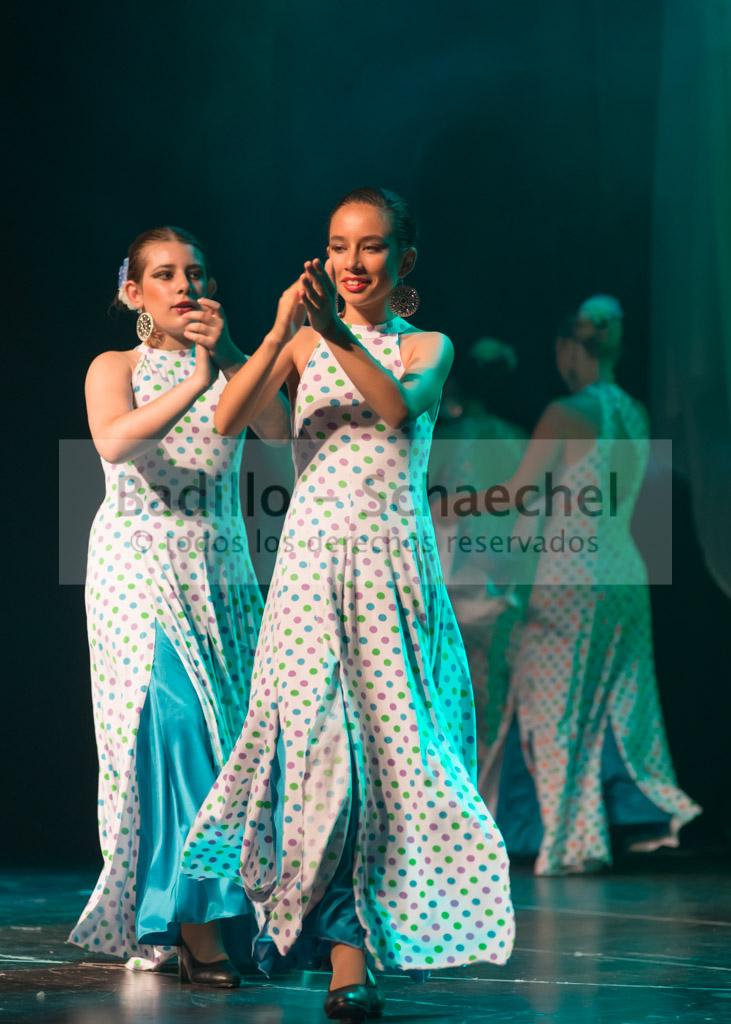In this detailed image, a group of young Latina girls, aged around 12 to 13, are lined up on a stage, seemingly participating in a beauty contest or performance. They are all dressed in the same sleeveless, ankle-length white dresses adorned with pink, lime, light blue, and purple polka dots. Beneath these dresses, a light purple layer peeks out. The girls are wearing matching black shoes and large gold earrings with intricate designs, contributing to their uniform appearance.

The stage itself is black, enhancing the brightness of their dresses. The focal point of the image is two centrally placed girls who are smiling, clapping, and perhaps dancing, creating a lively atmosphere. In the background, two more girls are partially visible, appearing to exit the stage.

A watermark text overlays the top of the image, reading "Badilo/Chanel shell" and "Todos Los Derechos Reservados," indicating all rights reserved in Spanish. This text, though slightly misprinted with variant spellings, marks the authenticity and copyrighted nature of the photograph.